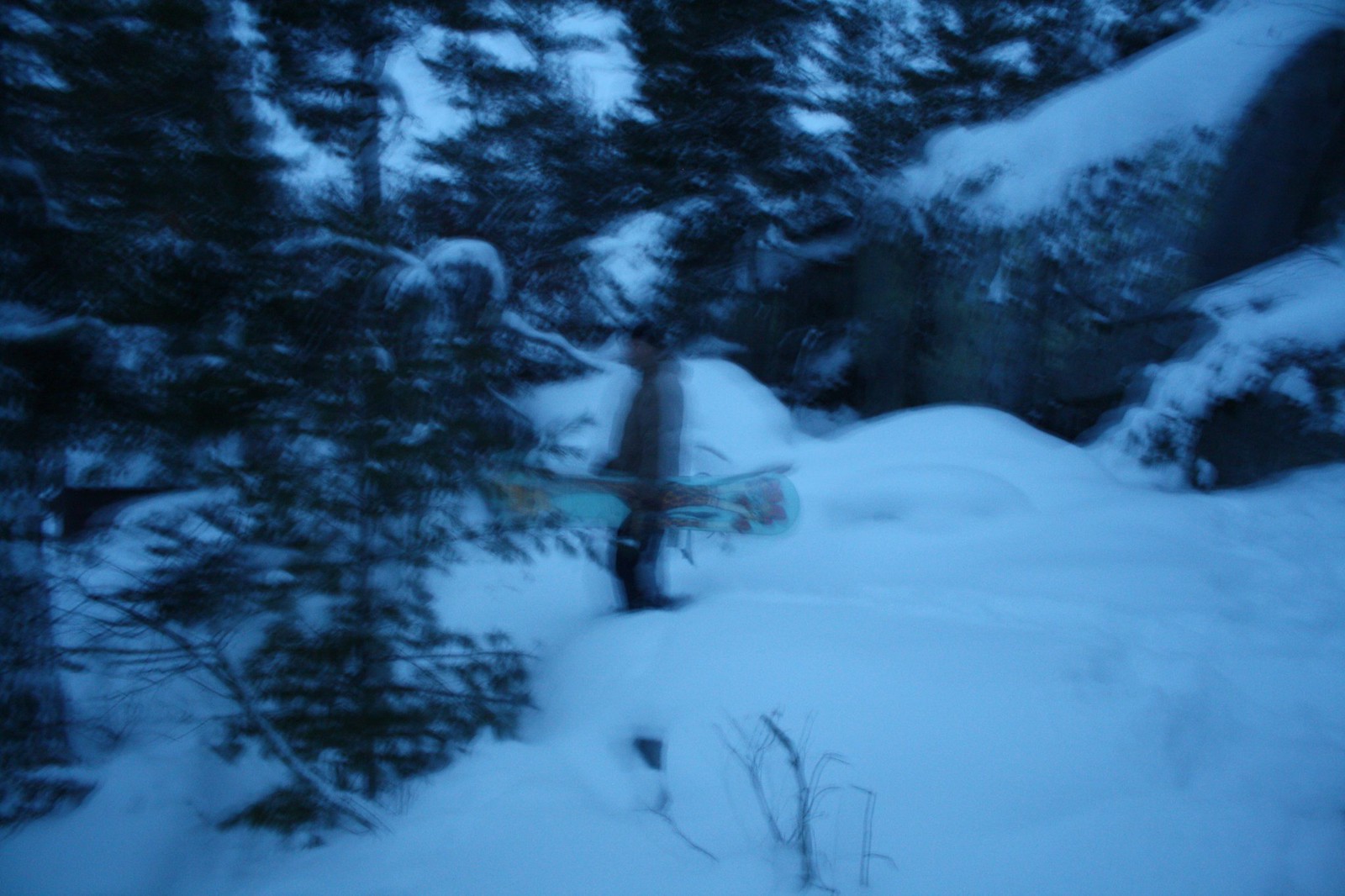In this image, we see a blurry and somewhat dark scene dominated by deep snow, creating a fuzzy, almost 3D effect. At the center of the picture stands a person, walking toward the left while wearing a cap, jacket, and long pants. The person seems to be holding something long, possibly a gun, though it is difficult to discern due to the blurriness. The image, which carries a blue tone mixed with black, suggests it might have been taken closer to nighttime. The lower right portion of the picture is filled with mounded snow, dotted with a few small branches. To the left, a group of evergreen trees laden with snow stretches up and across most of the upper part of the image. Near the upper right corner, there appears to be a large rock or dome-like structure with snow on top, giving an impression of a cave. The whole scene provides a wintry, slightly mystical atmosphere, capturing the rugged beauty of a snowy landscape.